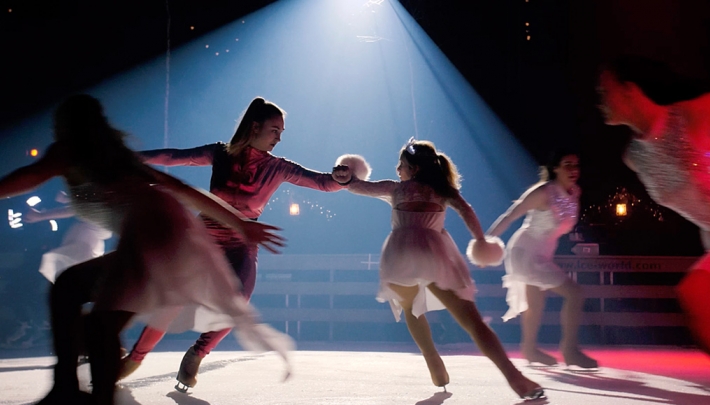The image captures a moment on an ice rink featuring six skaters engaged in an elegant routine beneath a central spotlight. In the foreground, a taller woman in a full-length scarlet red jumper and a young girl in a white ice-skating suit with furry cuffs are the focal points. They face each other, extending their arms to bump hands or forearms as they prepare to spin in unison. Surrounding them, four other skaters dressed in white and pink dresses or ballet-style uniforms glide softly, slightly blurred and outside the focus of the spotlight. The rink is enclosed by a white gate or barrier, providing a sense of containment within the larger darkened space. The spotlight casts a dramatic silhouette of the skaters against the ice, highlighting the grace and poise of their movements.